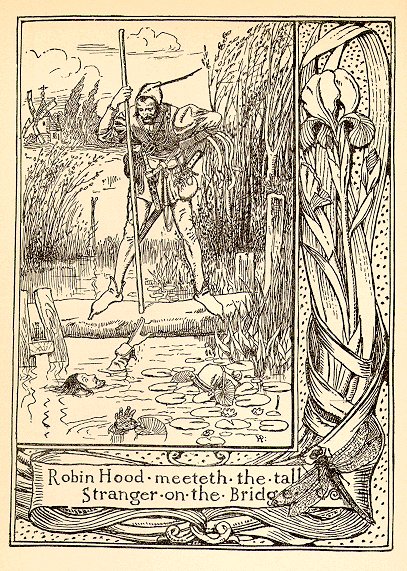This illustration, appearing on a yellowed page likely from an old, medieval-style book or pamphlet, portrays a dramatic scene involving Robin Hood. The black-and-white drawing features Robin Hood standing on a log bridge, with a peaked cap adorned with a feather. He has a large wooden pole in his right hand and a sword on his left. At the bottom of the page, the text reads "Robin Hood meeteth the tall stranger on the bridge." 

In the artwork, Robin Hood gazes down with a suspicious expression at a man who appears to be struggling in the water below, with his right hand reaching up towards Robin Hood. The scene is detailed with various elements: lily pads float on the water's surface, branches, and leaves from trees frame the right side, and a windmill is visible in the background on the upper left. The landscape includes grass in the distance and tall plants resembling wheat adorning the riverbank. Decorative flowers and a border embellish the lower and right sides of the page. The meticulous details in the illustration, including the man's floating hair and distressed facial expression, enhance the urgency and tension of the scene, raising questions about Robin Hood's next move—whether he will rescue the stranger or not.